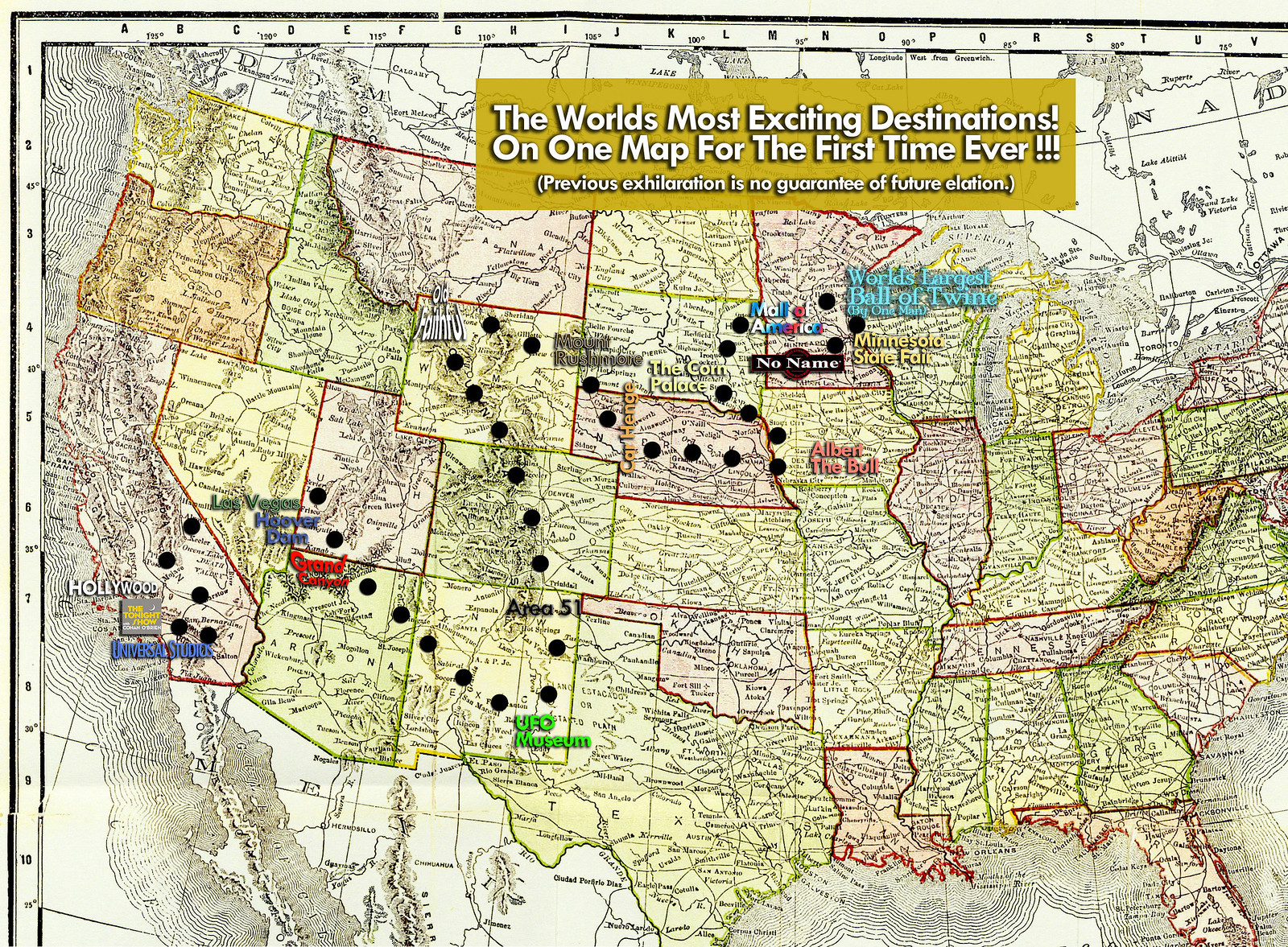This image depicts a detailed topographical map of the United States, highlighting elevation changes across the country. The map features numerous black circles tracing a route from Los Angeles to Las Vegas, proceeding through Phoenix, up to Salt Lake City, and eventually reaching Minnesota. Each state is outlined in red, with some states colored in yellow and others in white. The map includes a network of black and white lines representing highways and other key infrastructure.

Additionally, a golden box with white lettering at the top of the map reads, "The world's most exciting destinations on one map for the first time ever." Below, a cautionary note states, "Previous exhilaration is no guarantee of future exhilaration." In Minnesota, blue text marks the location of "the world's largest ball of twine," and yellow text highlights the "Minnesota State Fair."

Various other multi-colored annotations appear at the bottom of the map, adding further points of interest or notes. Notably, the state of Maine is cut off from the map, hinting at its primary focus on the central and western parts of the United States.